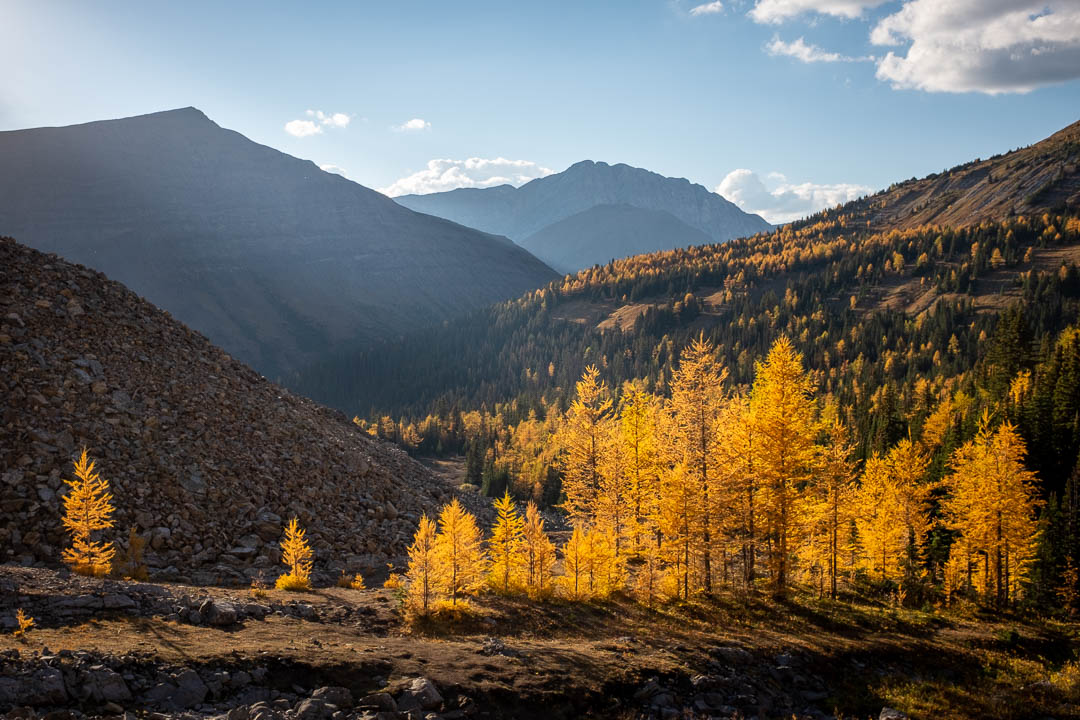The photograph captures a serene, sunlit outdoor landscape with a cascading series of hills and mountains, adorned with a spectrum of natural beauty. Dominating the center of the image are coniferous trees, boasting a golden glow, indicative of the fall season, with yellow leaves shimmering in the sunlight. In the foreground, the hills appear brown or dark grey and are covered in pebbles and gravel, adding a rugged texture to the scene. A meandering brown soil path carves its way through the landscape, inviting the eye to follow.

Above, a light blue sky, dotted with white clouds, stretches across the horizon, enhancing the tranquil ambiance. In the distance, a prominent blue mountain rises, its slopes transitioning into foothills that interlock with each other, creating a layered effect. These foothills also feature trees, contributing to the lush, verdant appearance of the region.

To the left of the image, a gravelly hill adds a contrasting roughness, while to the right, another hill, more heavily forested, balances the composition. The photograph exudes a calm and picturesque vibe, capturing the essence of a peaceful day in nature.